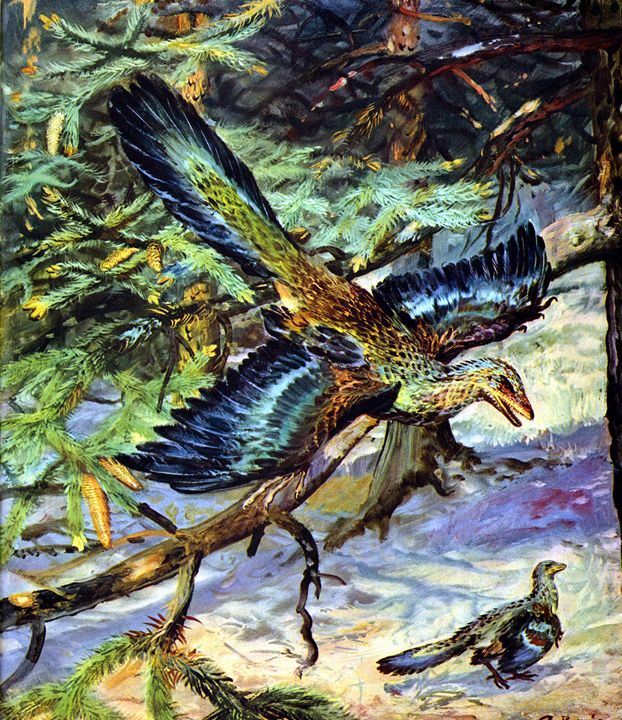The artwork is a vertically oriented painting depicting two fantastical bird-like creatures amidst an evergreen tree with intricate details. One creature is perched on the ground, showcasing a vibrant set of wings adorned with shades of blue, dark red, and light blue outlines. Its tail feathers are a striking combination of dark black and blue, while the mane and back display a greenish-yellow hue with scattered spots.

The second creature, reminiscent of a baby dinosaur with bird-like features, is perched on a branch in a top-down view. It has expansive, outstretched wings with dark blue feathers transitioning to light blue toward the tips, edged with black. Its body is greenish-tan moving towards dark black or blue tail feathers with blue undertones. This creature, poised as if about to take flight, has a lizard-like mouth instead of a beak, a narrow eye slit, and a thick neck leading to its bird-like body, adding to its prehistoric appearance.

The background features evergreen foliage with pine cones and an intricate network of branches. Notably, a large branch hangs prominently, contributing to the scene’s dynamic composition. The painting, rich in abstract elements, captures the surreal blend of avian and reptilian traits, bringing to life these unique, prehistoric-looking creatures in a vibrant, natural setting.